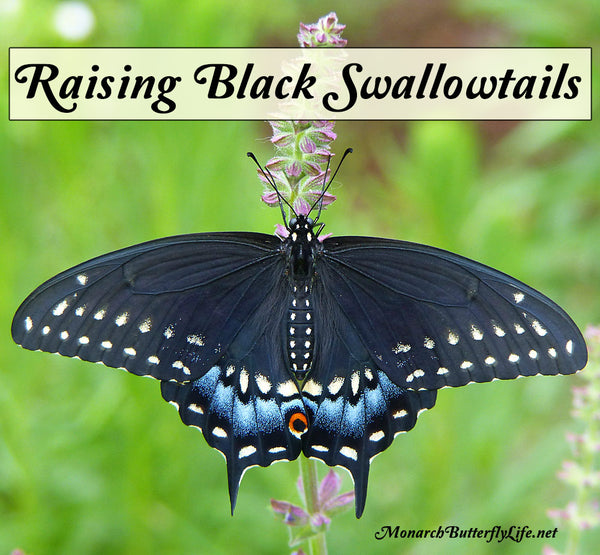The image captures a beautifully detailed close-up of a solid black Swallowtail butterfly, prominently titled "Raising Black Swallowtails" in a fancy black font at the top. The butterfly is perched on a tall stalk of a flower with a green stem and multiple pinkish-purple buds that have yet to bloom. The butterfly's open wings reveal intricate patterns: the upper wings are decorated with small off-white semicircular dots, while the lower wings showcase turquoise coloration speckled with white dots, and an orange dot with a black center. This elegant butterfly also features a distinctive two-pronged tail. The background is a lush, blurred green, enhancing the focus on the butterfly and flower. In the bottom right corner, the website monarchbutterflylife.net is subtly noted, adding a touch of informational reference to the serene and picturesque scene.